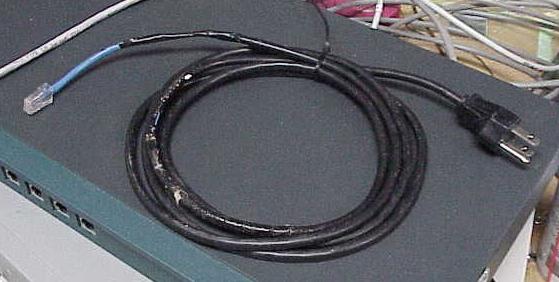This photograph features a close-up view of a network switch, typically used for connecting multiple devices within a network setup, such as in an office environment. The switch facilitates the allocation of network resources across various connected computers. For instance, in an office setting with five computers—one designated for video editing and the others for general office tasks—the network administrator could allocate more bandwidth (e.g., 300 MB of a hypothetical 500 MB network) to the video editing workstation to optimize its performance. The remaining bandwidth would be distributed among the other computers for routine tasks like email and web browsing.

In the foreground of the image, there is a visibly worn Ethernet cable, which appears to have been spliced. This cable has a blue wiring section terminating in a clear plastic RJ45 connector. Attached to it with electrical tape is a black wire that seems to be damaged, possibly gnawed or severed, leading to a standard power cord at its end. The photograph also shows an assortment of other cables, primarily dark gray and white, scattered on a light gray or tan table in the background. The overall scene suggests an improvised or makeshift networking setup, possibly in need of maintenance or upgrading.